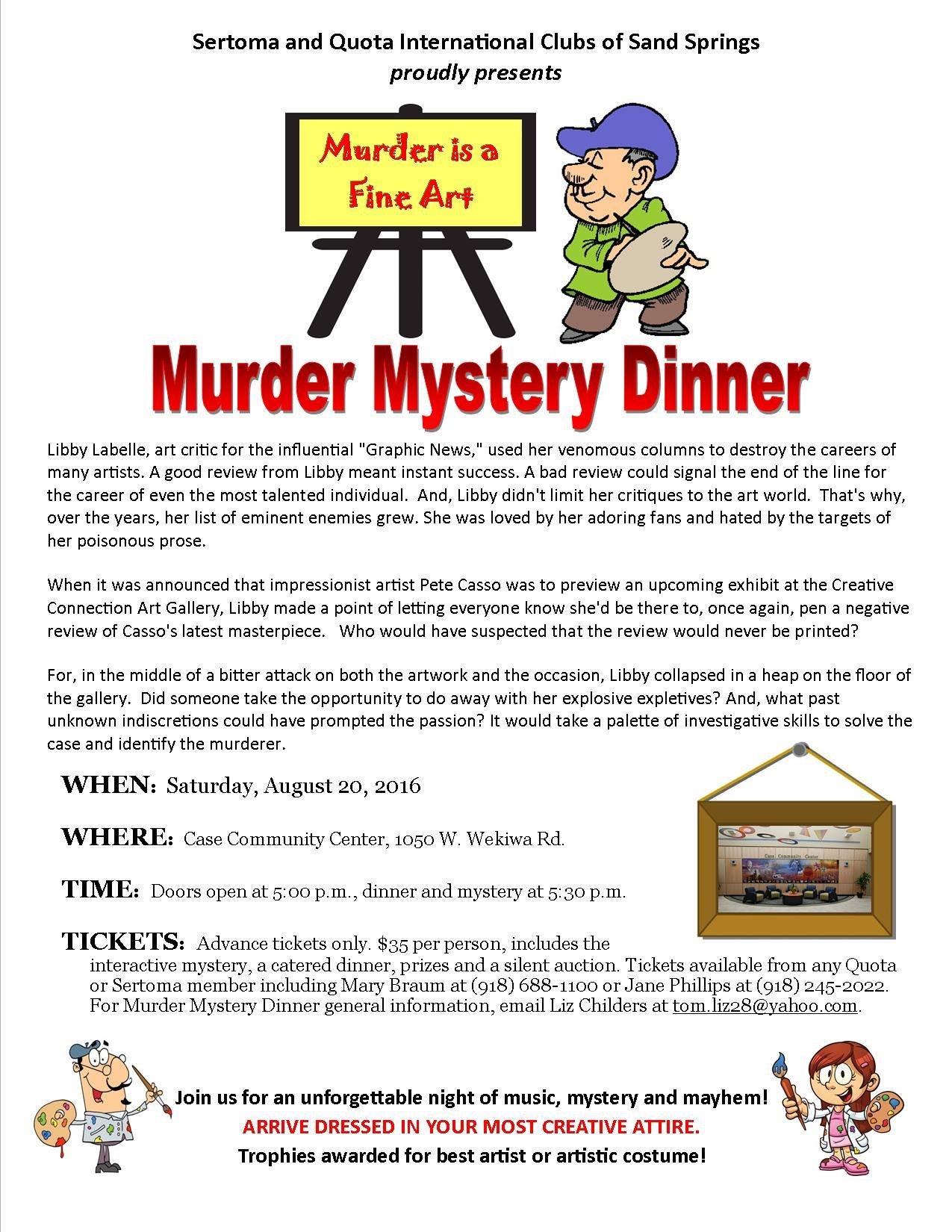Join us for an unforgettable night of music, mystery, and mayhem as the Sertoma and Quota International Clubs of Sand Springs proudly present a Murder Mystery Dinner titled "Murder Is a Fine Art." The event features a computer-generated advertisement with vivid details: at the top, "Serotoma and Quota International Clubs of Sand Springs proudly presents" is written in black. Below this, a clip art style image of an easel shows a painting that says, "murder is a fine art" in red on a yellow background, created by a small artist wearing a blue hat and a green shirt. In large red letters beneath this, the text reads, "Murder Mystery Dinner."

The storyline of the mystery centers around Libby Labelle, an art critic for the influential Graphic Times, known for her venomous columns that could make or break an artist's career. Her cutting critiques extended beyond the art world, earning her numerous enemies despite her adoring fanbase.

Details for the event are also present:
- **When:** Saturday, August 20th, 2016
- **Where:** Case Community Center, 1050 West Waikawa Road
- **Time:** Doors open at 5:00 PM, Dinner and Mystery begin at 5:30 PM
- **Tickets:** Advance tickets only $35 per person, available from any Quota or Sertoma member including Mary Baum at 918-688-1100 or Jane Phillips at 918-245-2022. For general information, you can email Liz Childers at tom.liz28@yahoo.com.

The night will include an interactive mystery, a specially catered dinner, prizes, and a silent auction. Arrive dressed in your most creative attire as trophies will be awarded for the best artistic costume. At the right side of the image, there's a small brown brand picture hanging with a string, adding to the overall artistic theme. At the bottom, it reads in black, "Join us for an unforgettable night of music, mystery, and mayhem" followed by, "Arrive dressed in your most creative attire" in red, and "Trophies awarded for the best artist or artistic costume" below that.